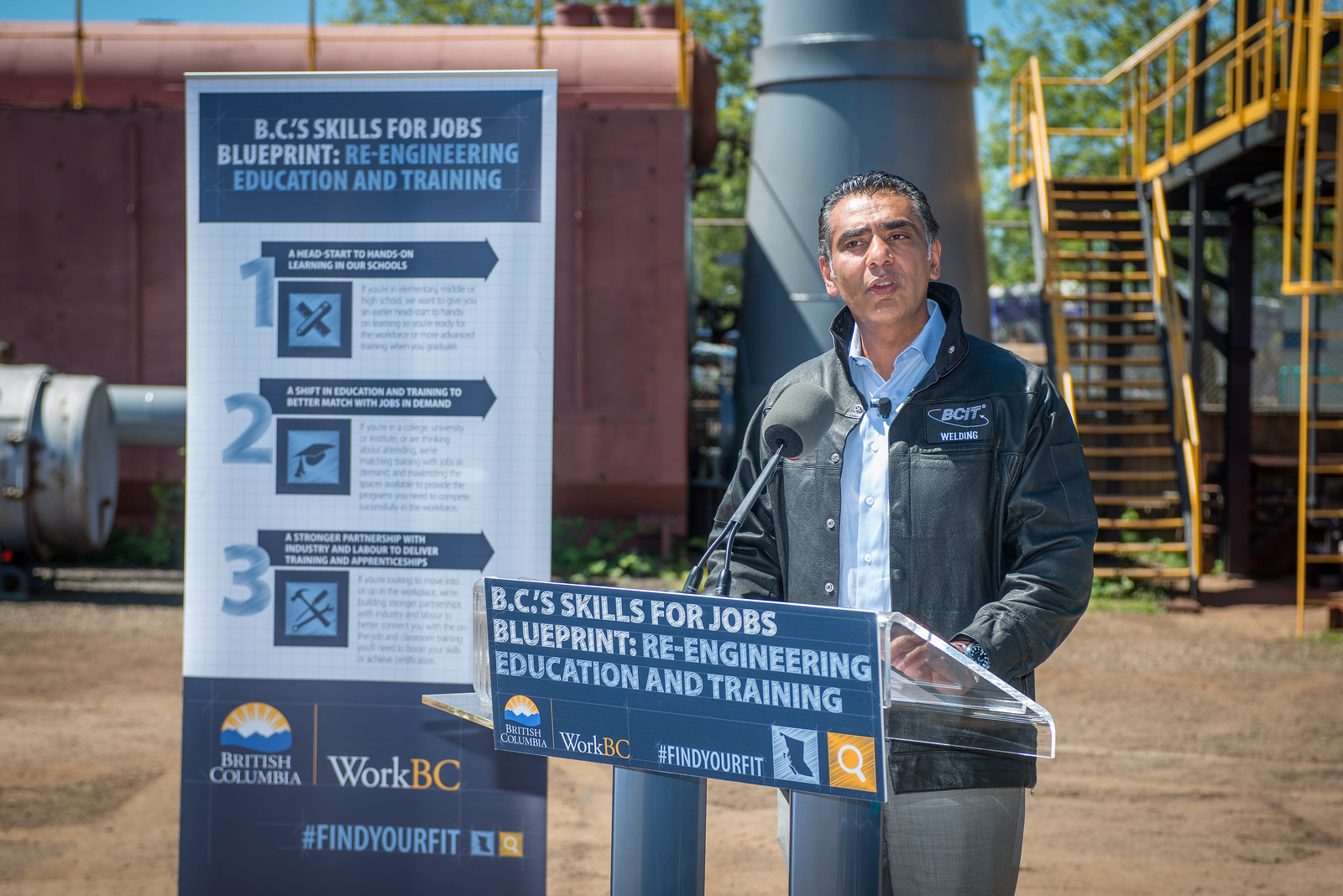In an image depicting an industrial setting with yellow railings and large metal machinery, a middle-aged man is seen speaking at a clear podium. The man, wearing a black bomber jacket with a BCIT welding logo and a light blue button-down shirt, is addressing an audience with a microphone pinned to his shirt. The podium features a blue sign reading "BC Skills for Jobs Blueprint: Re-Engineering Education and Training." Flanking him to the left is a large banner that echoes the podium's message and details three key points: "1. Head Start to Hands-On Learning in Our Schools, 2. A Shift in Education and Training to Better Match Jobs in Demand, and 3. A Stronger Partnership with Industry and Labor to Deliver Training and Apprenticeships." At the bottom of the banner, logos for British Columbia and Work BC are displayed alongside the tagline "#FindYourFit."